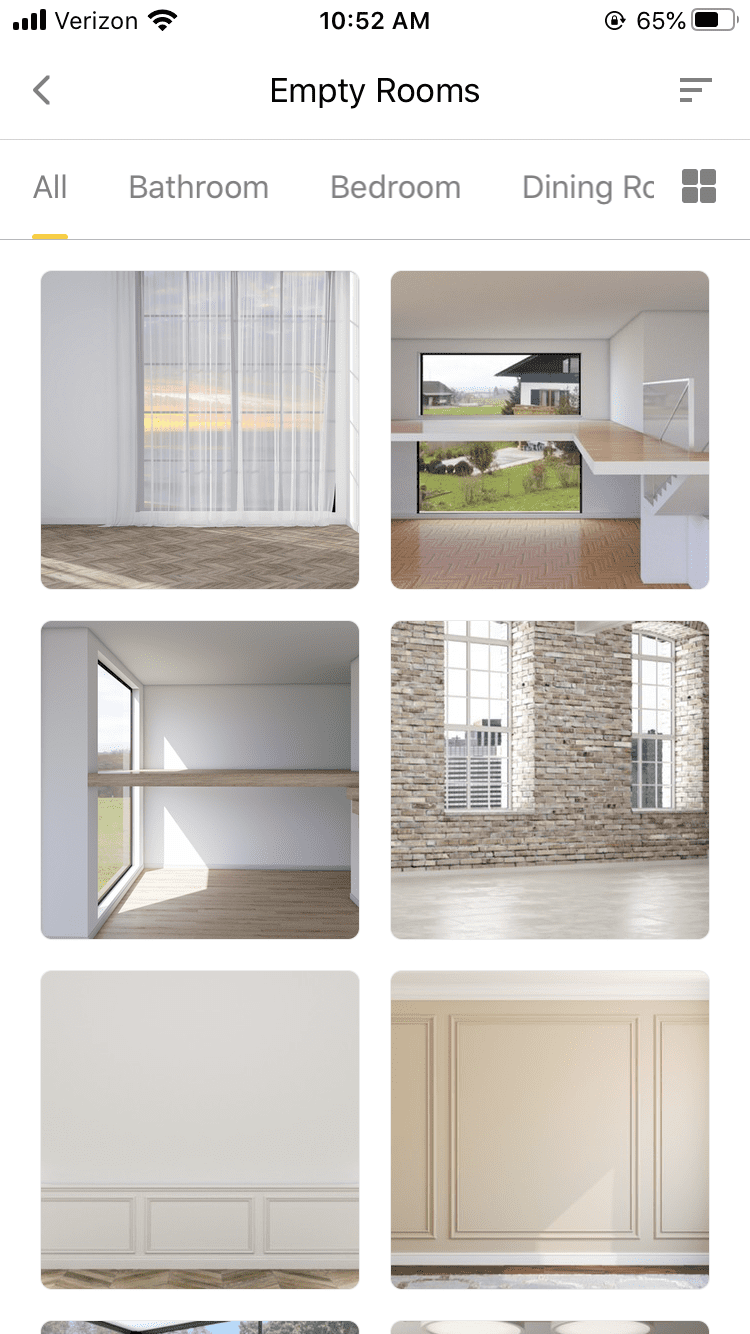This screenshot captures a detailed view of a smartphone interface. In the upper left-hand corner, the phone service carrier is displayed as Verizon, with a strong Wi-Fi connection indicated by all four bars being lit up. The time shown is 10:52 AM, and the battery life is at 65%. 

Prominently featured in the middle of the screen is the text "Empty Rooms," accompanied by navigational arrows on either side, allowing the user to scroll through options. Below the battery indicator, there are three horizontally aligned lines, implying a menu or settings option that can be accessed to refine the search further.

Continuing downward, the interface includes several tabs: "All," "Bathroom," "Bedroom," and "Dining Room." Notably, a yellow underline highlights the "All" tab, signifying that the current view is set to display all available information rather than information specific to a particular room. Additionally, there is a square icon comprised of four smaller squares, which likely provides access to more options when clicked.

At the bottom section of the screen, an image is visible, showcasing a nicely arranged patio with white sheer curtains and glossy brown hardwood floors. This image appears to be part of the content related to the "Empty Rooms" theme displayed above.